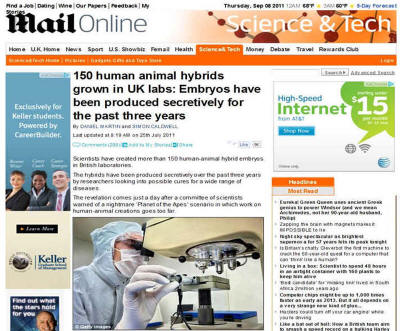This image is a somewhat blurry screenshot of a page from Mail Online, potentially associated with the Daily Mail. Dominating the top left is the Mail Online logo. On the right side of the header, "Science and Tech" is highlighted, indicating that this is the current section of the site. Below the header is a navigation bar featuring various categories, such as Home, UK Home, News, Sport, UK, Showbiz, US Showbiz, Health, Science and Tech (highlighted in orange), Money, Travel, and others partially obscured.

The main headline reads, "150 human-animal hybrids grown in UK labs", referencing secretive production over the past three years, ostensibly dating back to 2011. The source of this information is not clear. The article is accompanied by an image of a scientist examining something under a microscope.

The page is cluttered with various advertisements. On the left side, a blue ad is visible along with an ad for Keller. On the right side, there's an ad promoting high-speed internet service for $15. The overall blurry nature and small size make further details difficult to discern.